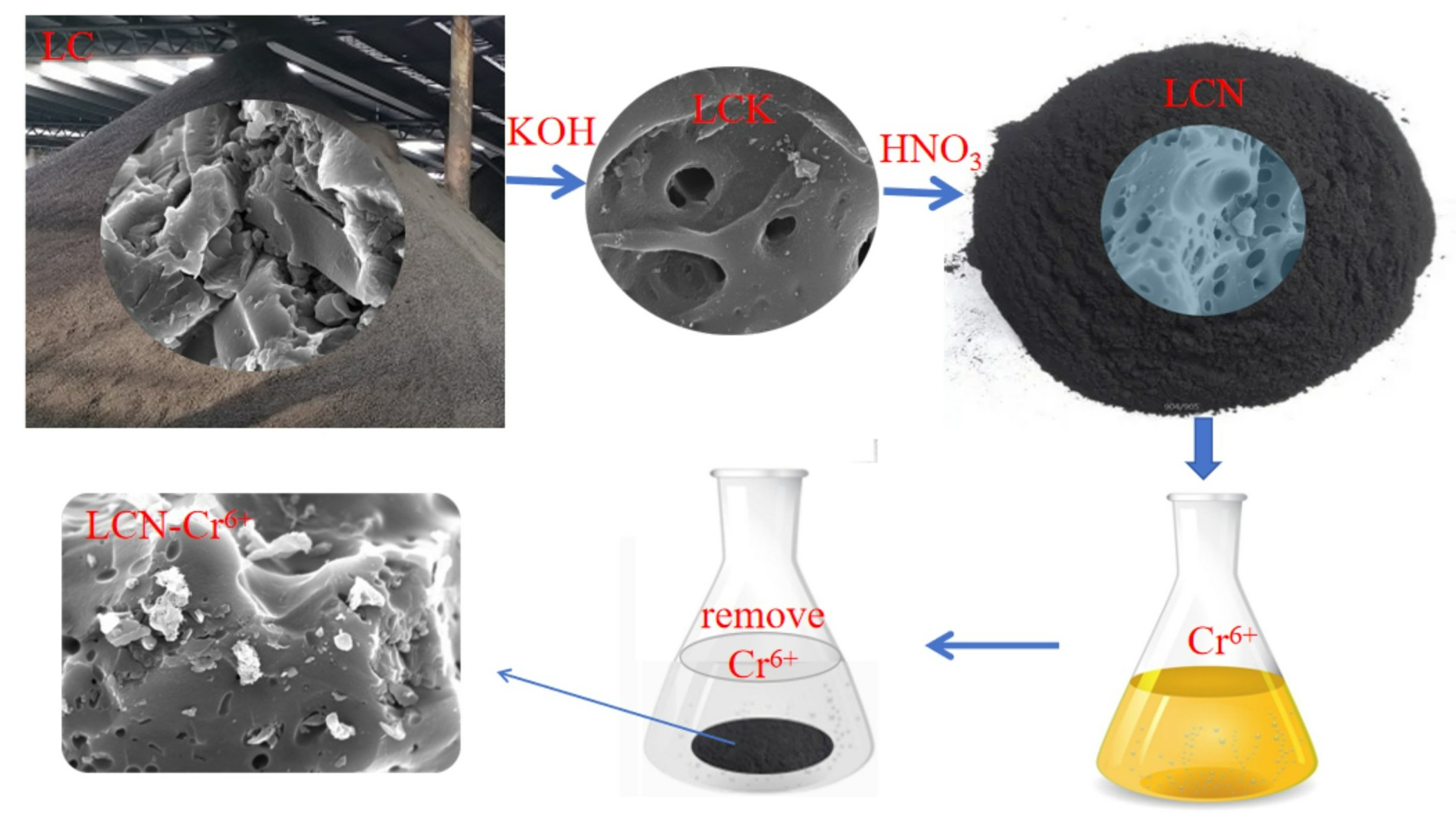The image is a detailed scientific flowchart illustrating a chemical process involving a mineral. It combines color photography with graphic design. In the landscape-oriented image, there are six photographs arranged in two rows of three. The two photos on the left depict a gray metal substance, with one showing the metal substance in a granular form. The center of the top row features arrows and chemical labels such as "Elsie", "KOH", "Elsie K", "HNO", and a noticeable gray circle with a charcoal-like rim and blue detail. 

The bottom row starts with a label "LCNCR" and includes beakers labeled "remove CR 6+" and "CR 6+". The beakers contain yellow fluid. The flowchart uses blue arrows and red text to indicate the chemical transitions and processes. Additionally, the bottom right image shows a close-up of the altered mineral or rock. The style blends realism in the color photography with illustrative elements to effectively convey the scientific context.